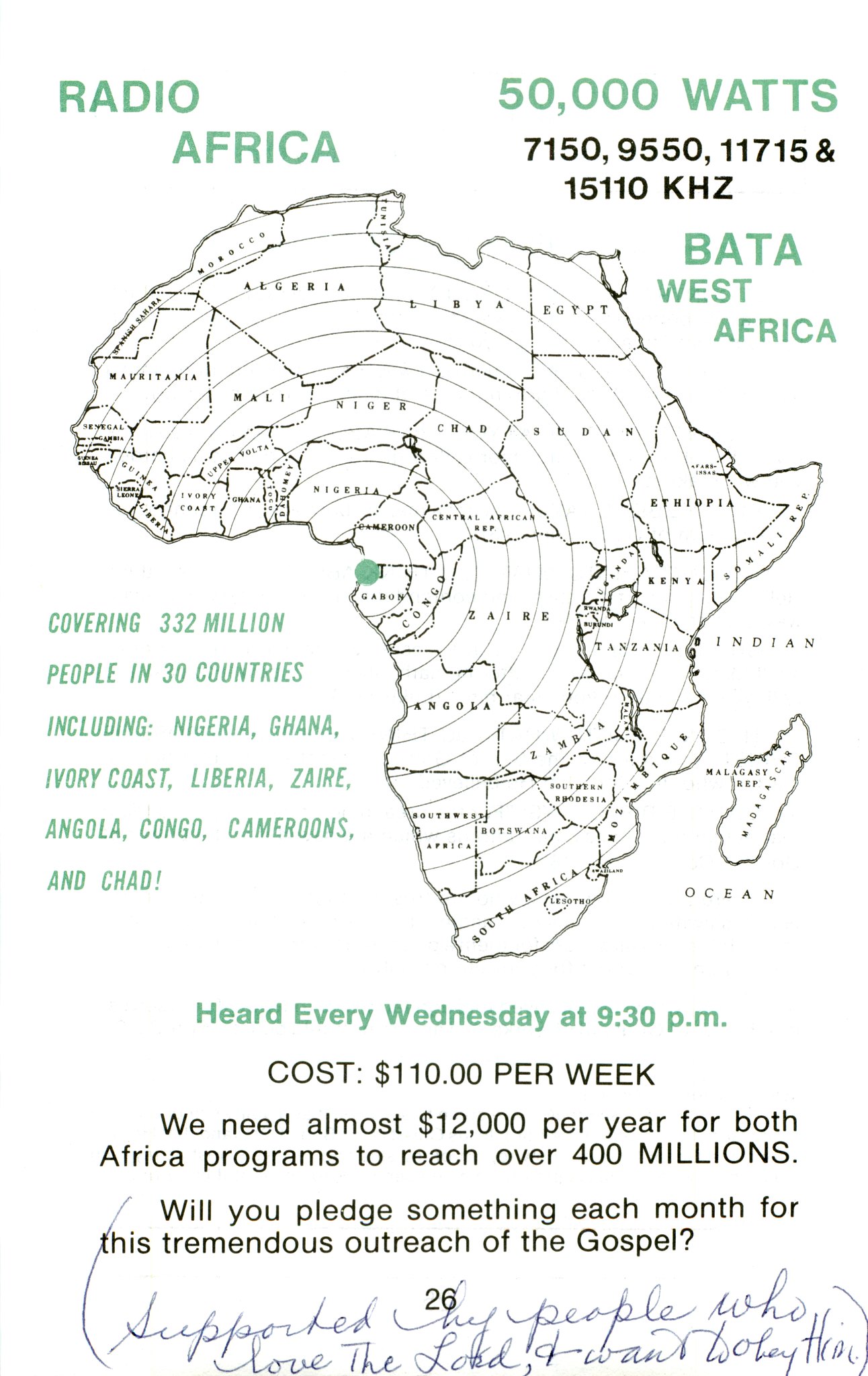This advertisement for Radio Africa is set against a white background. Dominating the image is an intricately detailed map of Africa, with every country clearly labeled. From a green dot near Gabon on the western coast, numerous concentric circles emanate outward, symbolizing radio waves covering the continent. In the top left corner, in uppercase green letters, it reads "Radio Africa." Adjacent to this, on the right, it states "50,000 watts" and lists specific frequencies: 7,150; 9,550; 11,715; and 15,110 kHz. Below, it mentions "Bata, West Africa." 

Midway to the left of the map, green text proclaims, "Covering 332 million people in 30 countries, including Nigeria, Ghana, Ivory Coast, Liberia, Zaire, Angola, Congo, Cameroons, and Chad." Beneath the map, it indicates the broadcast schedule: "Heard every Wednesday at 9:30 p.m." followed by the cost: "$110 per week." Further, it appeals for financial support: "We need almost $12,000 per year for both Africa programs to reach over 40 million. Will you pledge something each month for this tremendous outreach of the gospel?" The number "26" is noted below in black, with a handwritten note in cursive stating, "Supported by people who love the Lord and want to obey Him."